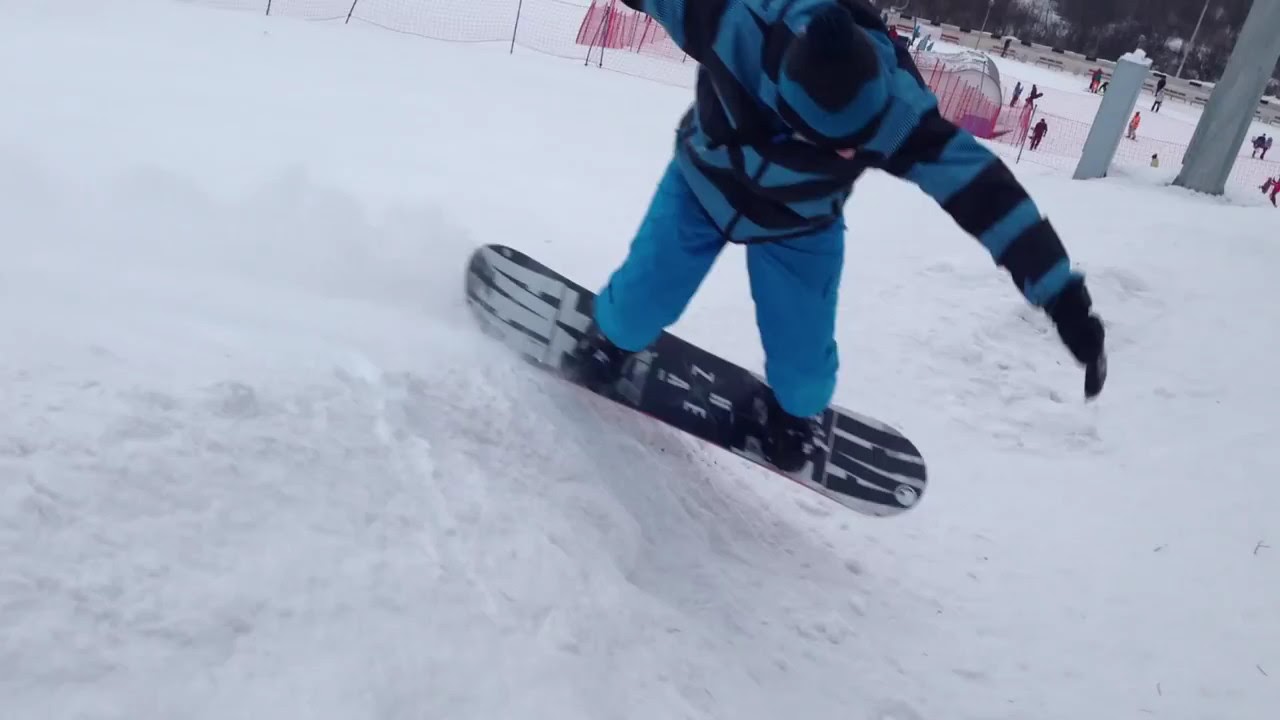In this vibrant outdoor photograph set on an expansive ski run, a snowboarder takes center stage, soaring midair just after clearing a snow-covered hump. The snowboarder, dressed in a matching ensemble of blue pants and a black-and-blue striped jacket, is captured in mid-flight with their body angled downward, emphasizing the thrill and skill of their jump. The figure's face is obscured as they look down, adding an element of mystery. They wear black gloves and a blue and black knit cap, complementing their slick, coordinated outfit. The snowboard beneath them is a sleek mix of gray and black. The backdrop showcases a snowy expanse dotted with fencing, posts, and several other individuals either walking or skating on the snow. Additionally, a line of woods can be seen farther back, framing the energetic scene with a touch of nature. The photo vividly depicts the excitement and dynamic atmosphere of the snowboarding experience.